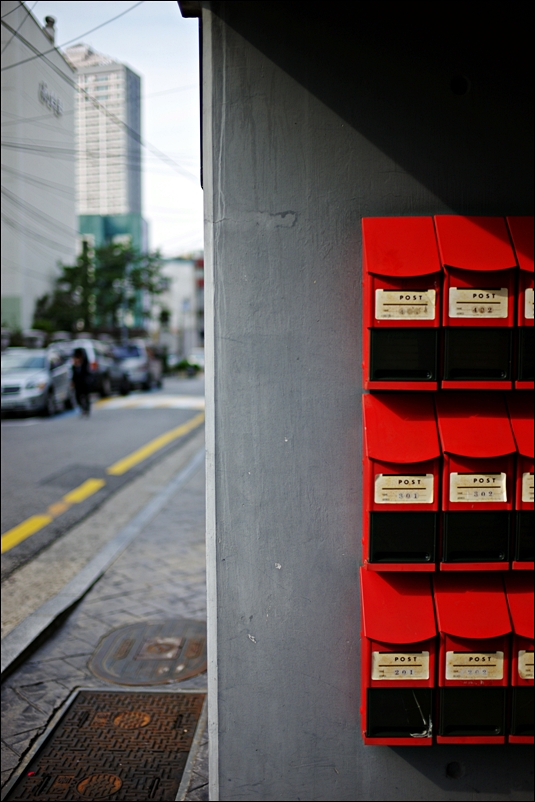This photograph captures the outer vestibule of a building featuring an array of bright cherry red post boxes, tightly arranged in a grid pattern on a gray, concrete-like wall. The right side of the image, occupying approximately 60% of the frame, showcases three rows of these post boxes, stacked three high and closely aligned both horizontally and vertically. Each post box is equipped with a slanted lid designed for mail deposit, angled around 40 degrees, and displays a white sticker with the word "POST" in bold black letters, followed by a series of three-digit apartment numbers, although the specifics are somewhat blurred.

To the left of the post box array, the scene transitions into a cityscape visible through an open doorway. This portion of the image reveals a blurry sidewalk and street receding into the background, with parked cars, large distant buildings, and a few indistinct figures. The street is marked with a yellow line, metal plates are embedded in the sidewalk, and overhead phone lines stretch across the scene, completing the urban setting.